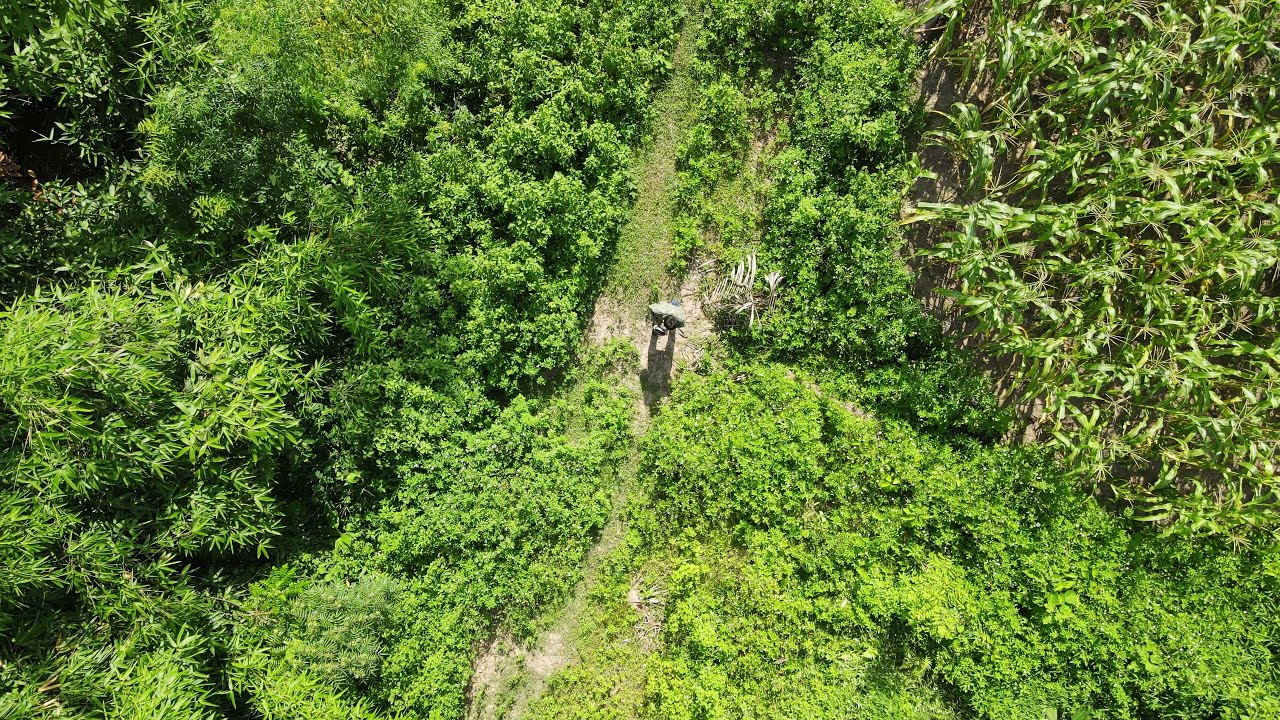This overhead aerial photograph captures a vibrant, sunlit nature area teeming with various shades of green foliage. The image, taken from a bird's-eye view, showcases an expanse of trees, bushes, and grass, ranging from dark to bright yellowish-green hues. Among the vegetation, the leaves are diverse: some trees have bushy or floppy canopies, while others feature thick, short, or slender, pointy leaves. Dominating the center of the image is a figure that initially appears to blend into the landscape but can be distinguished by a person-shaped shadow cast on a patch of exposed brown dirt. The person, who seems to be wearing green, is surrounded by plants that resemble tall crops, possibly corn stalks, though the exact species is hard to discern from the height at which the photo was taken.